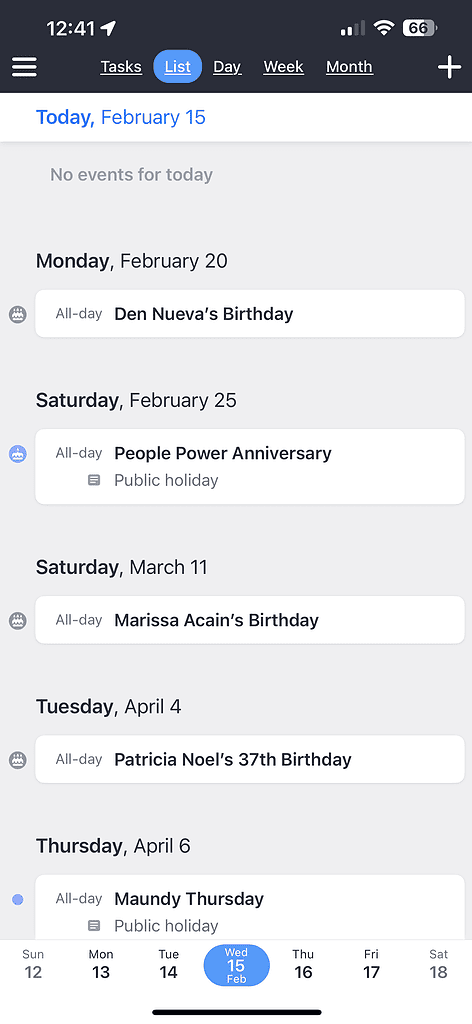**Screenshot of a Phone's Calendar App on February 15th**

The screenshot captures the phone's calendar interface on Wednesday, February 15th, at 12:41 PM. The phone is in airplane mode, with Wi-Fi enabled and showing two bars of signal strength. The battery level is at 66%. A three-line context menu icon is located in the upper left-hand corner.

The calendar features a black background with contrasting white text. The main section is titled "Tasks," with a blue background highlighting the selected "Lists" tab. Adjacent tabs, "Day," "Week," and "Month," are displayed in black. A plus icon on the far right allows adding new events.

The immediate view displays a gray background with segmented white rectangular bubbles for each listed event. The daily agenda for upcoming days includes:

- **Monday, February 20th:** Geneva Duneva's birthday (all-day)
- **Saturday, February 25th:** People Power Anniversary, a public holiday (all-day)
- **Saturday, March 11th:** Marissa R. King's birthday (all-day)
- **Tuesday, April 4th:** Patricia Noel's 37th birthday (all-day)
- **Thursday, April 6th:** Mondrian Thirsty, a public holiday (all-day)

At the bottom, the calendar shows dates for the week including Sunday, the 12th to Saturday, the 18th of February.

This well-detailed calendar screenshot provides an overview of scheduled events and birthdays, organized in an intuitive and user-friendly design.